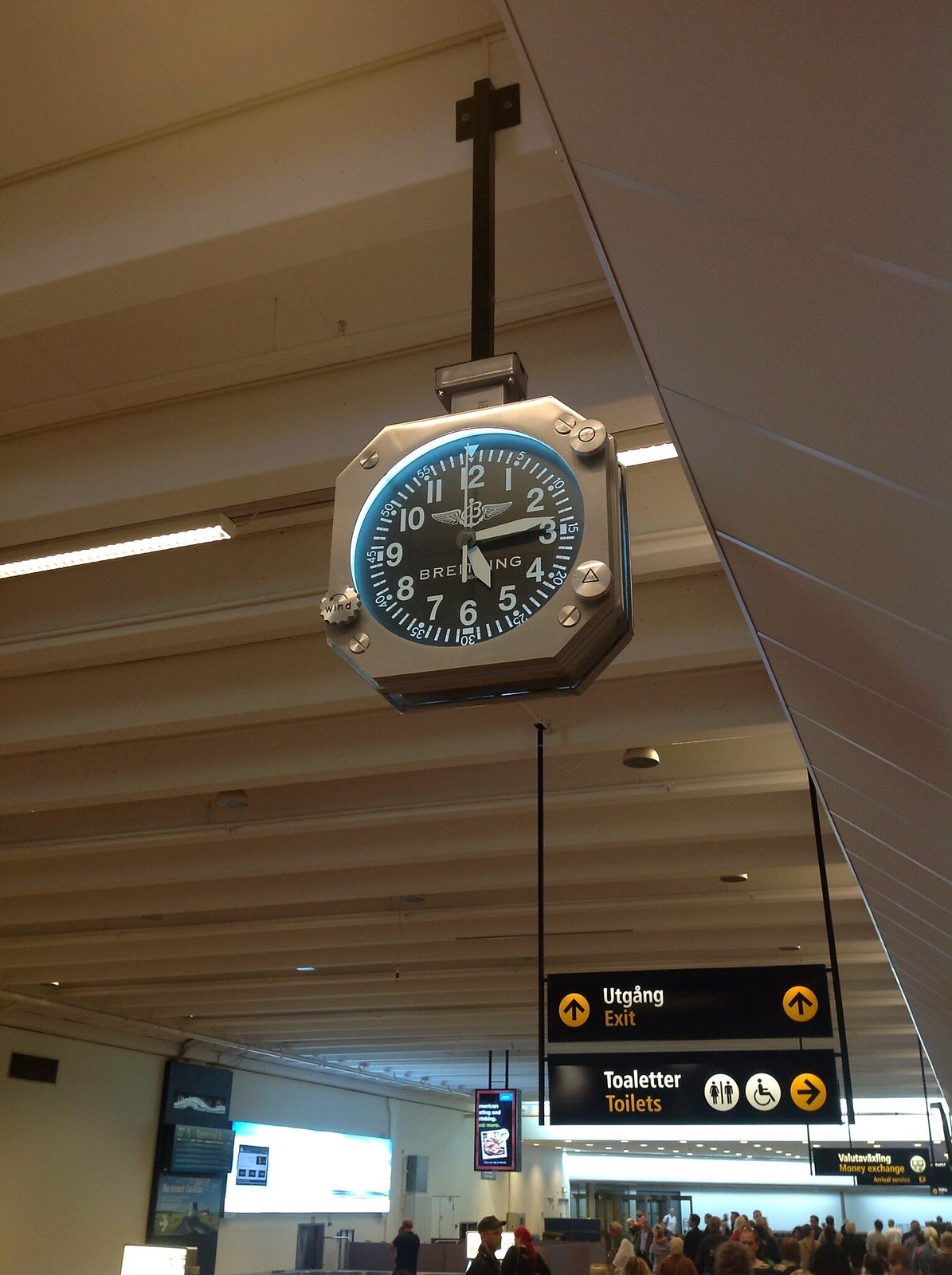This image depicts a clock affixed to the ceiling of a transportation hub, likely an airport or bus station. The off-white, possibly beige ceiling features tiered panels extending downward, possibly for acoustic purposes, giving it a distinctive texture. Prominently displayed in the foreground is an octagonal clock with a sleek silver frame. The clock face is a striking black adorned with white Arabic numerals, showing the time as approximately 5:14. Surrounding the clock face are metal buttons, adding a functional aesthetic. A black rod supports the clock, securing it to the ceiling.

In the background, there are directional signs hanging from the ceiling. The upper sign reads "Utgang" and "Exit," while the lower one reads "Toileter" and "Toilets," each accompanied by arrows pointing towards the respective facilities. The scene is populated with around 20 to 30 individuals, who appear to be waiting for their next mode of transportation.